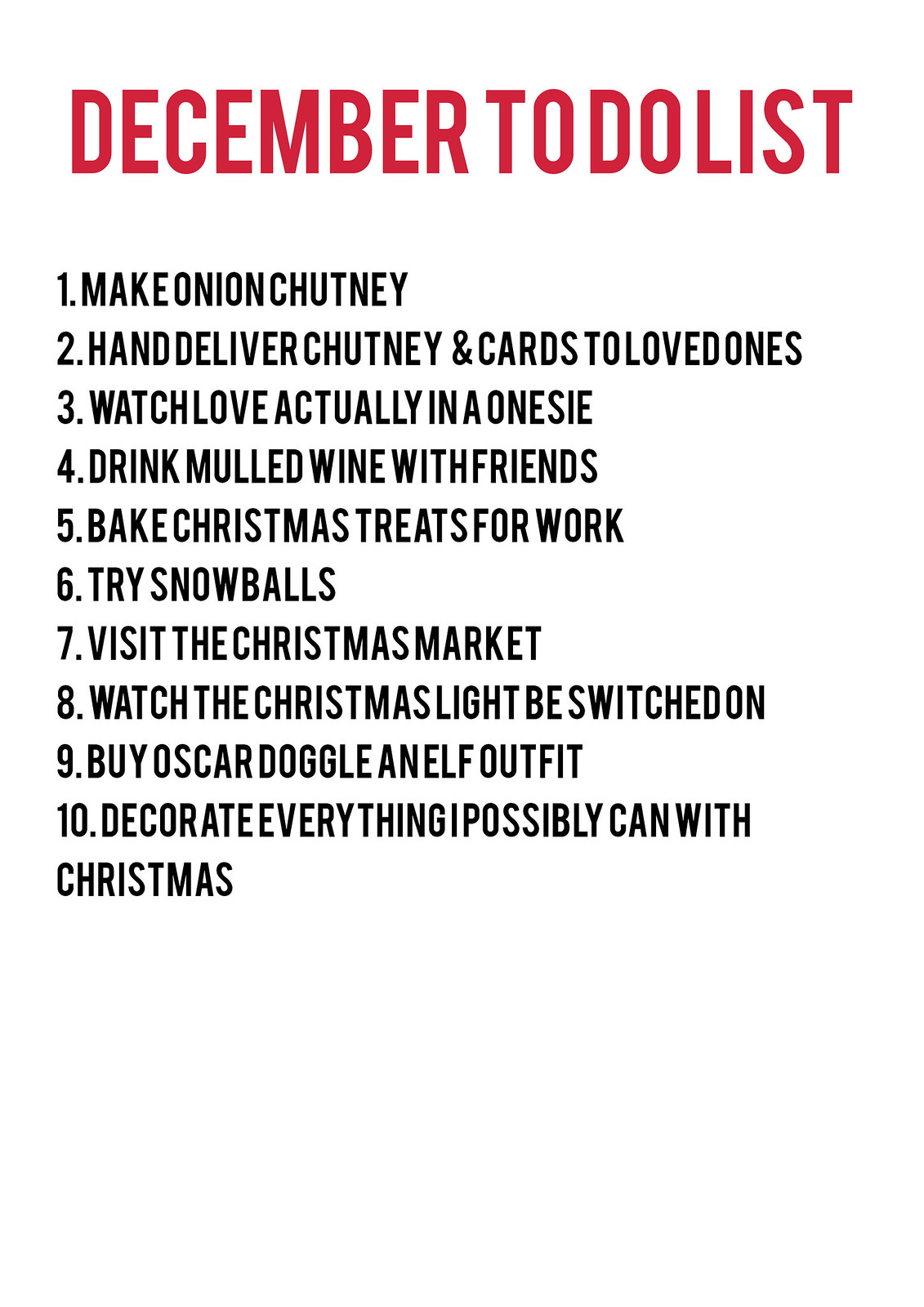The image is a December to-do list with a stark white background. At the top, in large, bold red capital letters, it reads "DECEMBER TO-DO LIST." Below this heading, there are ten numbered tasks listed in black capital letters, each without any space after the period before the text. The tasks are: 

1. MAKE ONION CHUTNEY 
2. HAND DELIVER CHUTNEY AND CARDS TO LOVED ONES 
3. WATCH LOVE ACTUALLY IN A ONESIE 
4. DRINK MULLED WINE WITH FRIENDS 
5. BAKE CHRISTMAS TREATS FOR WORK 
6. TRY SNOWBALLS 
7. VISIT THE CHRISTMAS MARKET 
8. WATCH THE CHRISTMAS LIGHT BE SWITCHED ON 
9. BUY OSCAR DOG A ELF OUTFIT 
10. DECORATE EVERYTHING I POSSIBLY CAN WITH CHRISTMAS

The only colors in the image are red and black, emphasizing the simple yet festive nature of the list.